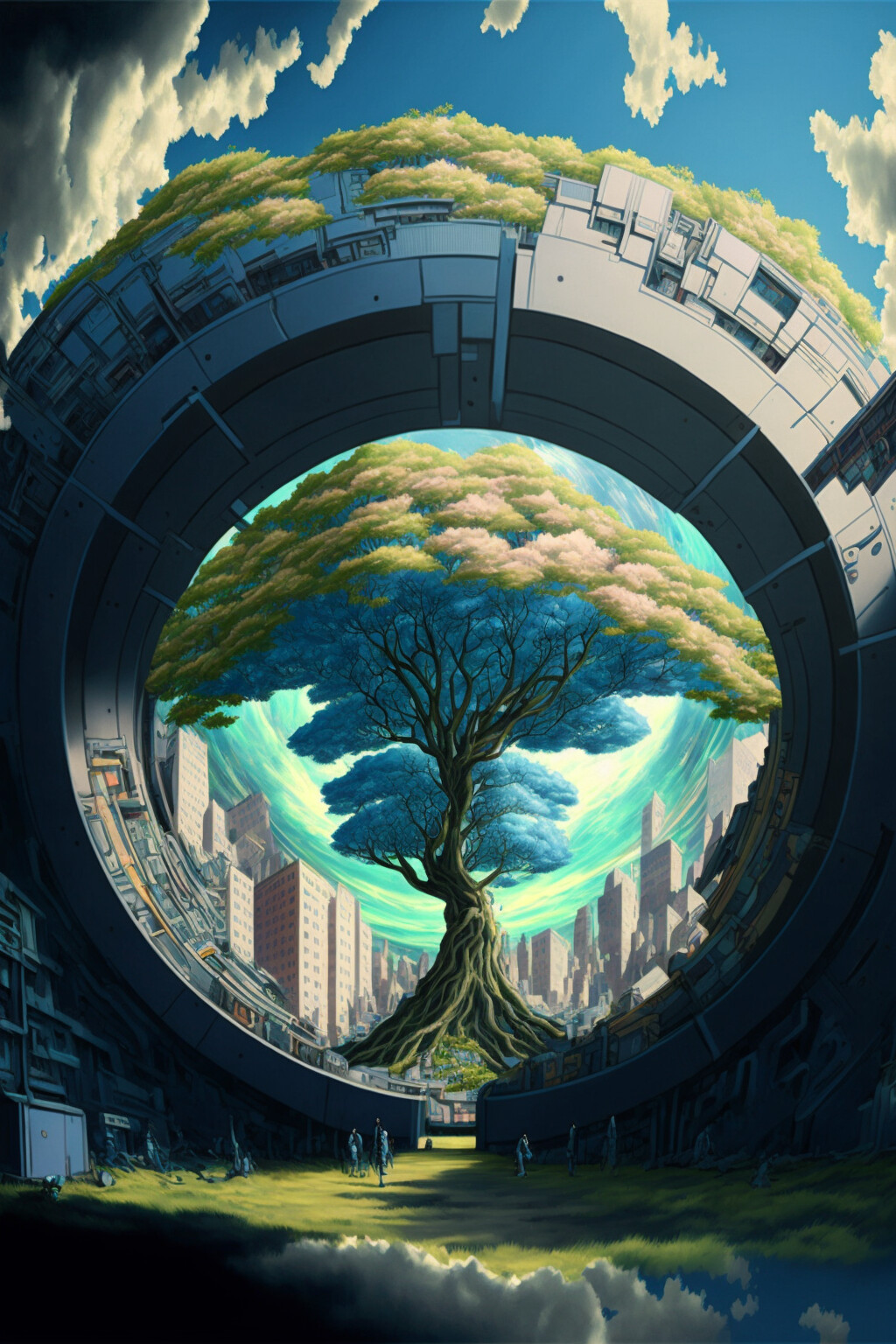The image is a detailed computer-generated digital artwork of a futuristic city floating in the sky. Surrounding the city is a massive, circular ring of intricate machinery that appears to keep it airborne. At the heart of this aerial city lies a striking circular gateway, framing a grand tree whose vibrant roots extend beyond the gateway structure. The tree's branches exhibit a blue hue near the bottom, transitioning into lush green and pink foliage that towers above the gateway. Encompassing the tree and the gateway are high-rise buildings arranged in a sweeping arc. Below, people stroll on the verdant grass, seemingly captivated by the majestic centerpiece. The backdrop reveals a skyline with a blue sky and scattered white clouds, enhancing the ethereal atmosphere of the floating metropolis.